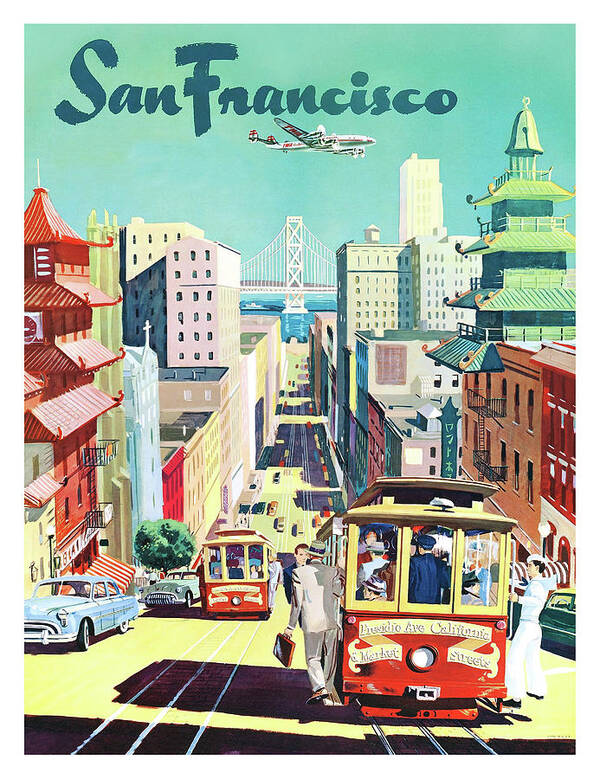This vibrant vintage travel poster from the late 1940s to mid-1950s beautifully captures the bustling streets of San Francisco. The poster is in portrait orientation, with a striking turquoise sky at the top, featuring the name "San Francisco" in an elegant black cursive script. Below the text, a propeller airplane soars from left to right.

The foreground is dominated by a red and yellow trolley car emblazoned with "Presidio Avenue." Passengers include Navy men in white uniforms and businessmen in suits. The street is lined with vintage 1950s automobiles, including a big sedan like a Chevy parked on the left side. The lively streetscape features a mix of architecture, from high-rise office buildings to iconic pagoda-style structures—one red on the left and a taller green one with multiple tiers on the right. 

In the background, the white towers of the Golden Gate Bridge stand majestically over the blue waters of the bay, adding an iconic touch to the scene. The entire composition exudes a sense of nostalgia and a rich historical ambiance, making it an excellent representation of mid-century San Francisco.